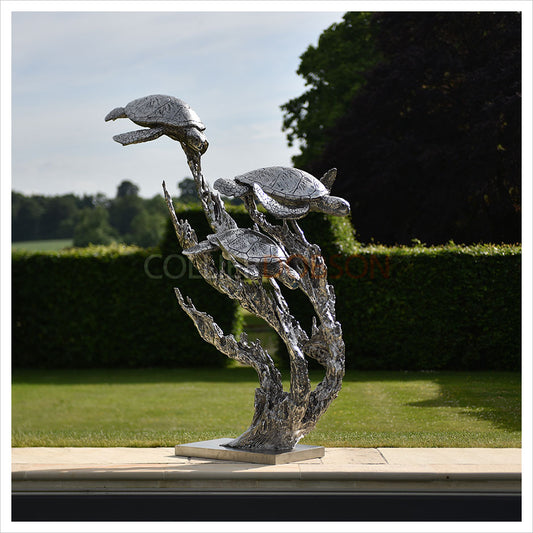The photograph, taken outdoors on a sunny day with a few clouds dotting the sky, captures an artistic silver-colored sculpture of three realistic-looking sea turtles swimming amidst curvaceous, flowy structures designed to resemble plants, coral, or seagrasses. The turtles, with their fins prominently displayed, are arranged as if they are heading towards the right and slightly downward, while the surrounding metal fronds curve to the left, creating an elegant flow. The entire sculpture rests on a white or silver rectangular base, which in turn is perched atop a stone ledge or small cement wall. The scene is set against a lush backdrop featuring a manicured green lawn, well-maintained hedges, and several vibrant green trees. The upper portion of the image reveals the blue sky, enhancing the overall tranquil and picturesque atmosphere. There is also an unreadable watermark running across the center of the image.